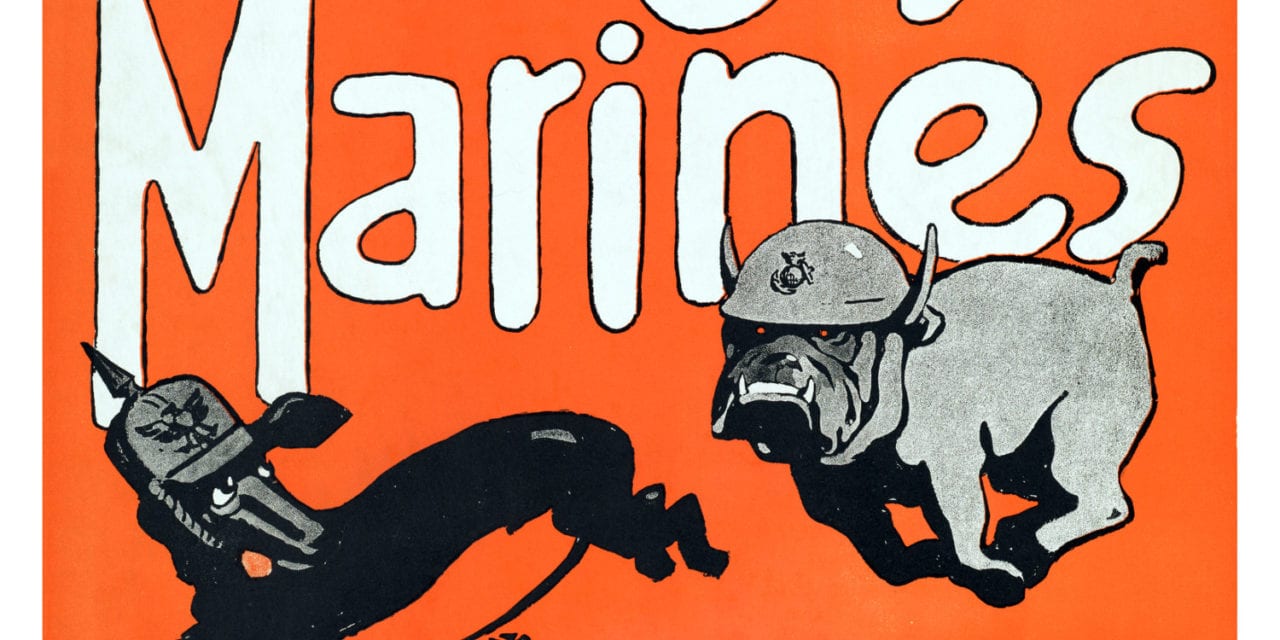The image is a vintage poster featuring an orange background and large white text that prominently reads "MARINES." This text spans across the top half, with some other text above it appearing partially cut off. The focal point below the text is the dynamic scene of two dogs in mid-chase: a black dachshund and a gray bulldog. The black dachshund, depicted as a long and lean dog with a long snout, is running while looking back with wide, fearful eyes. This dachshund is wearing a helmet featuring a protruding spear, evoking the image of a German soldier. Chasing it is a muscular gray bulldog with a menacing expression, red eyes, and exposed, intimidating teeth. The bulldog, bearing a hard helmet reminiscent of a U.S. Army helmet, is depicted with a tail, unlike the tail-less dachshund. This intense chase, combined with the militaristic symbolism, suggests it is a propagandistic piece aimed at evoking nationalist sentiments.